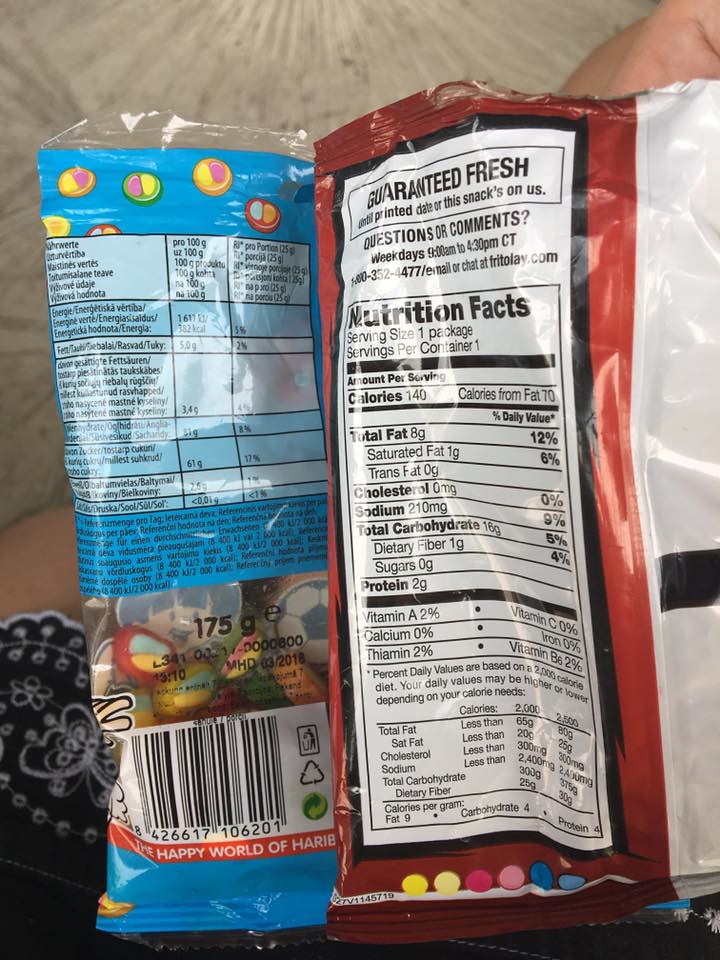In the photograph, we see the back of two snack packages held by a person. The left package is a blue Haribo candy bag, adorned with images of green, pink, and yellow candy pieces along the top. The bag features nutritional information in another language, showing it contains 175 grams of candy. A barcode and a recyclable symbol are also visible, along with the tagline "Happy World of Haribo." The right package appears to be the back of a small, red Doritos bag. It prominently displays nutritional facts, including 140 calories per serving, 8 grams of total fat, and 2 grams of protein, with other details like "Guaranteed Fresh," a contact number, and a website. The person holding the packages is wearing a black floral shirt with white butterfly stitching, and their left arm is extended, while their right hand, assumed to be holding the Doritos bag, isn't visible. The background reveals a room with concrete walls and a design, suggesting a casual, indoor setting.